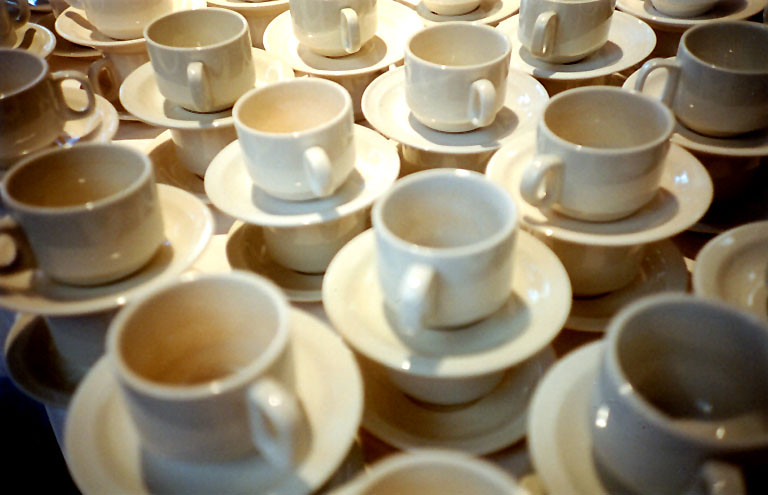The photograph captures a tightly composed scene featuring numerous white ceramic coffee cups stacked on matching white saucers. The cups, reminiscent of those found in cafeterias or catering companies, are organized in multiple rows that fill the entire frame, with at least six visible rows oriented diagonally. Each row is stacked two to three layers high, creating a sense of depth and repetition. The lighting is harsh, emanating from the upper middle of the image, casting shadows and radiating reflections on the glazed surfaces of the cups and saucers. This interplay of light and shadow results in varying tones across the image, from lighter highlights to darker areas, particularly noticeable in the lower left-hand corner. The cups are uniformly styled and feature small handles suitable for one or two fingers, designed to hold approximately 10 ounces of liquid. The image is cropping tightly around these rows, leaving no other elements visible, focusing all attention on the orderly arrangement of the cups and saucers.